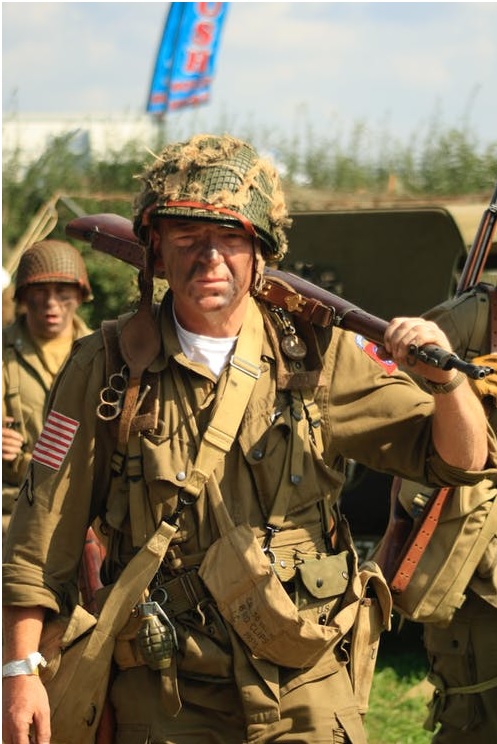The photograph captures a poignant scene of a World War II reenactment featuring three men in military uniforms. The central figure, who is the main focus, stands facing the camera with a neutral expression, his face marked with black paint camouflage. He wears a tan uniform, a green helmet with netting and burlap straps, and a wristwatch on his right hand. His uniform is detailed with numerous pouches, straps, and brass knuckles on a shoulder pad, and he carries a brown rifled gun slung over his left shoulder. An American flag patch adorns his right arm, while a red flag is on his left arm. To his left, another man in an olive drab uniform and helmet appears struck or possibly having Down syndrome; his helmet is similarly netted. On the right, partially obscured, is another man, identifiable only by his carrying bag, leather strap with rivet holes, and a gun. The background reveals a modern setting, with a blue and red Busch beer sign and what appears to be a sky of light grayish-blue tones, confirming that this is indeed a reenactment. The scene blends historical authenticity with contemporary elements, making for a striking and immersive depiction of wartime remembrance.